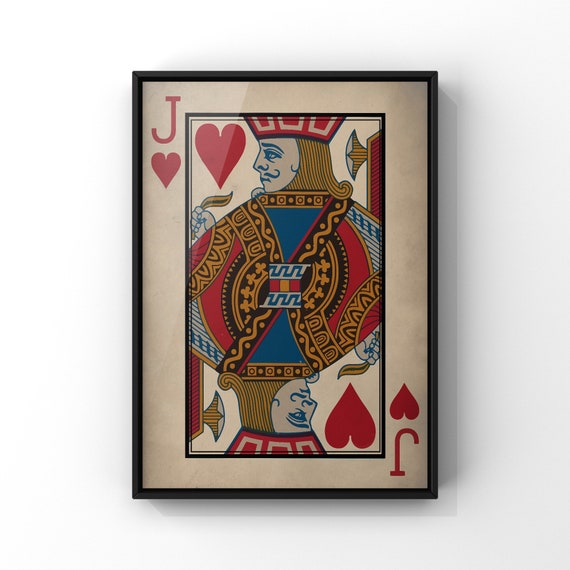The image features a framed Jack of Hearts playing card set against a white background. The frame is a slim black one, housing a large, blown-up version of the card, which appears to be slightly weathered, giving it a bone-white color. The Jack of Hearts, with its vibrant red, gold, and blue attire, is depicted with a red crown and blonde hair. At the top left and bottom right corners, the card showcases the iconic red 'J' and heart symbols. The card is designed in the classic playing card format, with a mirrored image of the Jack's head and torso at the top and bottom. The card appears to be behind some sort of protective covering, possibly plexiglass or real glass, which adds to its preserved, keepsake appearance.